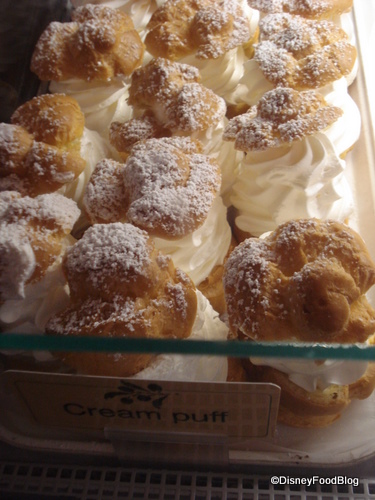The image depicts an enticing array of nine cream puffs meticulously arranged in a display case at a bakery. Captured from a slightly top-down angle, the photograph showcases the cream puffs through a clear, likely glass, casing. Each cream puff is crafted with a puffy, golden-brown pastry base and top, both generously sprinkled with powdered sugar. In between, there is a layer of luscious, cream-colored whipped cream, forming a delicate sandwich. The display is structured into three columns of three cream puffs each, neatly positioned on a tray. In front of the glass case, a horizontal beige cream-colored sign with black text spells out "Cream Puffs." At the bottom right corner of the image is a watermark that reads "Disney Food Blog" with a copyright symbol, denoted in white text outlined in black.